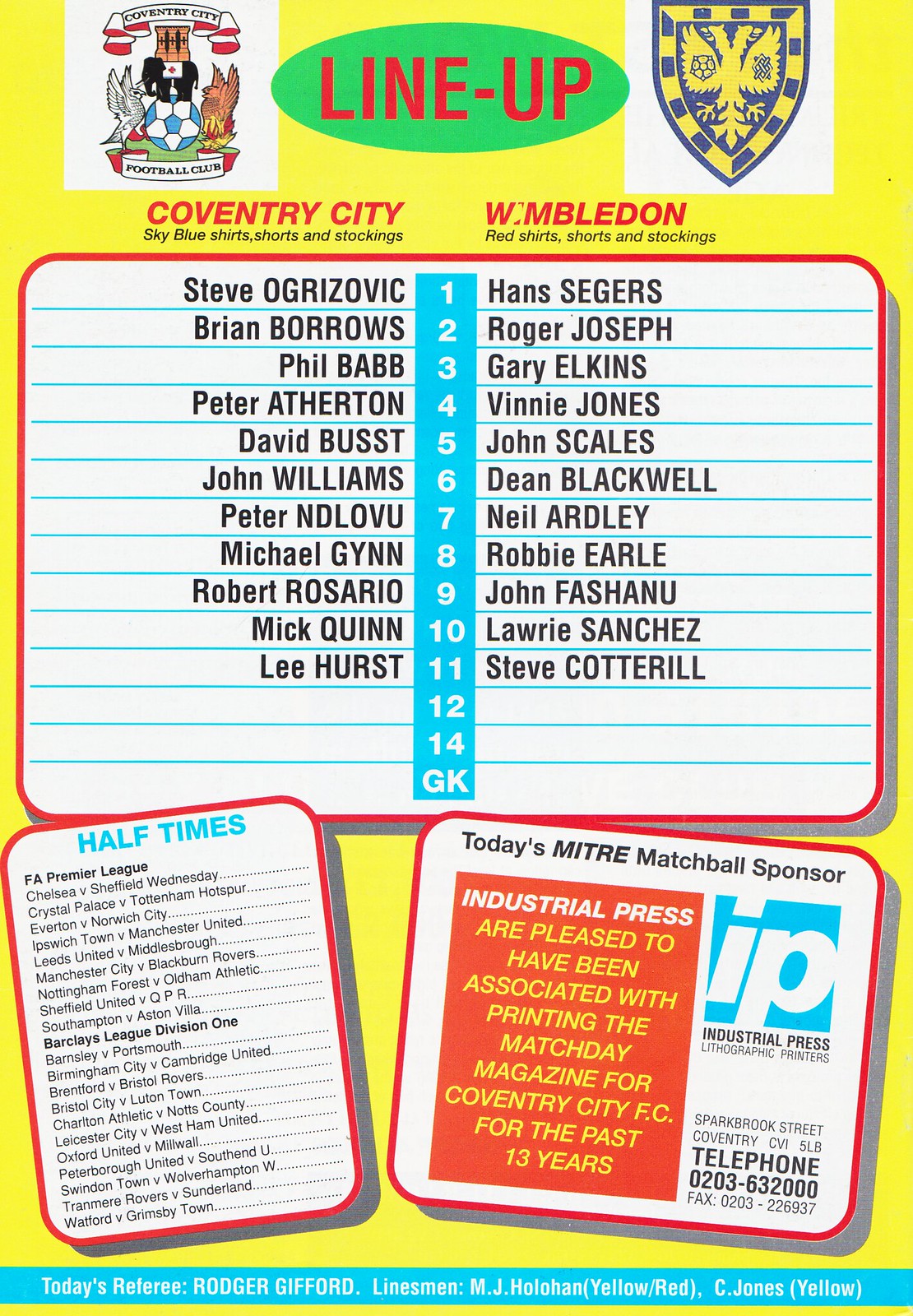The image is a sports program page with a bright yellow background. At the top left is the emblem of Coventry City Football Club, featuring a soccer ball, an elephant, a dove, and a griffin. On the top right is a shield with a yellow and blue background, possibly depicting a two-headed bird, representing Wimbledon. Between these emblems is a green oval with red text that reads "Line Up."

Below this, the left side in red states: "Coventry City Sky Blue Shirts, Shorts, and Stockings," while the right side in red states: "Wimbledon Red Shirts, Shorts, and Stockings." Under this, there's a white square resembling lined paper, with lines of blue. Running vertically down the center is a blue rectangle with white numbers ranging from 1 to 14. On the left side, it lists the names of Coventry players: Steve Ogrizovic, Brian Burroughs, Phil Babb, Peter Atherton, David Bust, John Williams, Peter Ndlovu, Michael Ginn, Robert Rosario, Mick Quinn, and Lee Hurst. On the right side are the names of the Wimbledon players: Hans Segers, Roger Joseph, Gary Elkins, Vinnie Jones, John Scales, Dean Blackwell, Neil Ardley, Robbie Earle, John Fashanu, Laurie Sanchez, and Steve Cotterell.

Below the player information, there are details about halftime events. At the bottom right is an advertisement for the sponsor, which reads: "Industrial Press Lithographic Printers, Sparkbrook Street, Coventry CVI, 5LB, telephone 0203-632-000, fax 0203-226937." Additionally, it mentions that Industrial Press has been pleased to be associated with printing the Match Day magazine for Coventry City FC for the past 13 years. At the bottom, the referee and linesmen are listed: "Today's referee: Roger Gifford, Linesmen: M.J. Hollowhand and C. Jones."